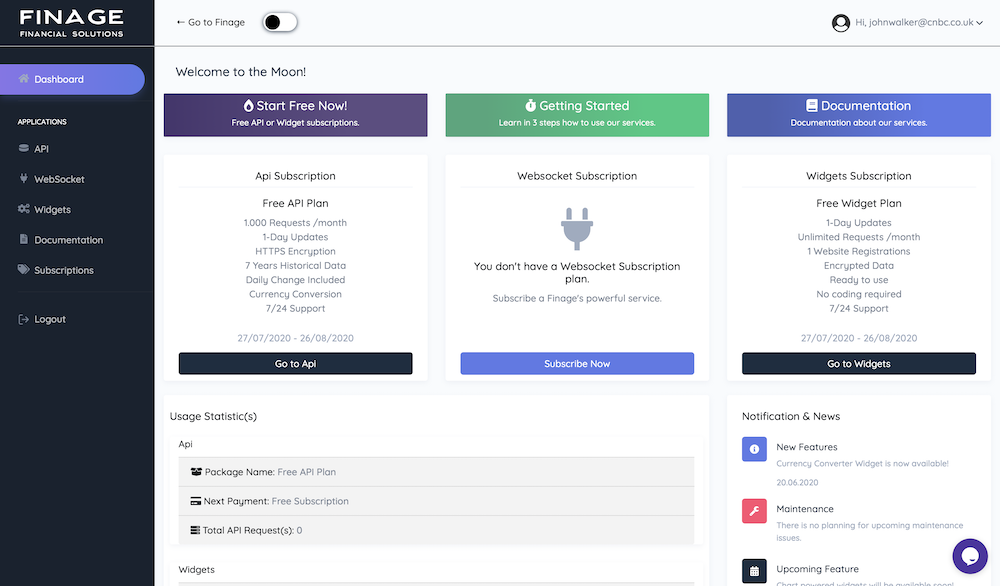The image depicts a web page with a predominantly white background. On the left-hand side, there is a prominent vertical black rectangle. At the top of this rectangle, the text reads "Finage, Financial Solutions," accompanied by a "Go to Finage" button. Below that, there's a small circular icon featuring a generic person figure next to the greeting "Hi". The name "John Walker" is mentioned, although his picture is not displayed.

The web page is divided into three sections or columns. The first section begins with a purple "Start Free Now" button. Below it, a green "Getting Started" button is present, followed by a blue "Documentation" button. Further down, this section contains a black "Go to Apple, Appy" button and a blue "Subscribe Now" button.

The second section highlights a black "Go to Widgets" button, maintaining the consistency of the white background that spans the entire webpage.